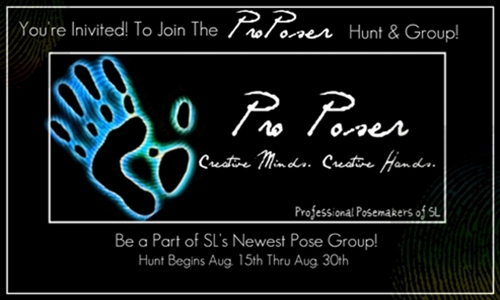"This image resembles a business card and features a predominantly black background. At the top, in white text, it proclaims 'You're invited to join the Pro Poser Hunt and Group!' Below this, in the center, is a white-bordered rectangle housing a pastel-colored, aura-like human handprint. Next to the handprint, the card reads 'Pro Poser' in a highly stylized and somewhat difficult-to-read script. Smaller text within the rectangle includes phrases like 'Professional Pose Makers of SL' and 'Be a part of SL's newest pose group.' At the bottom, more white text states, 'Hunt begins August 15th through August 30th.' The card is intricately detailed despite its minimal color palette, conveying an invite to a specific event related to pose making in a perhaps virtual or niche community known by the acronym SL."